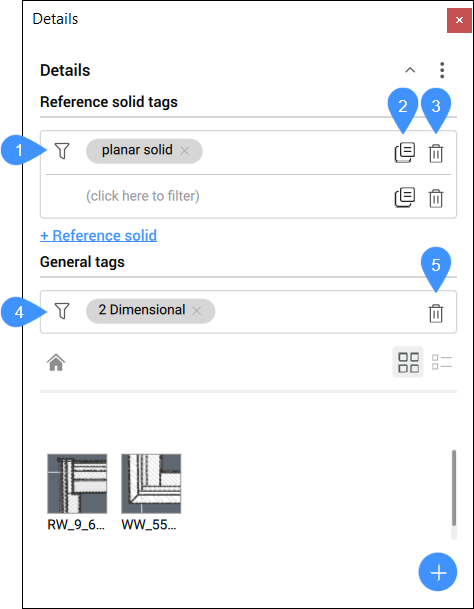This image is a vertical screenshot taken from a computer smart device, likely showcasing a user interface of some software. The background appears to be the user's computer screen with minimal detailing, giving the image a clean and professional look. 

At the top left corner, the word "Details" is displayed, adjacent to a deep red box with a white "X" inside, serving as a close button. Just below "Details," the word is repeated in bold, indicating it might be a section title. Beneath this, "Reference Solid Tags" is also displayed in bold, followed by a horizontal line that separates it from the following content.

The section underneath lists various items labeled as "Planar Solid," accompanied by a grey background and an "X" symbol. Several icons are displayed on this background, each with corresponding annotations:
- A trash can icon with the number "3" above it.
- A notepad icon with the number "2" inside a blue teardrop.
- An unidentified icon in front of "Planar Solid," with the number "1" inside a blue teardrop.

Adjacent to "Planar Solid," you can see an option to reference "Solid" in blue text and "General Tags" depicted in black text. An icon with the number "4" precedes these tags. Following this, "Two-dimensional" is mentioned alongside:
- A trash can icon with the number "5" above it.

Further down, there's a home icon, and finally, the string "RW96WW_55 Pictures," followed by a plus sign at the bottom of the section.

Overall, this detailed screenshot appears to be part of a larger user interface, potentially for managing or editing graphical or textual elements.